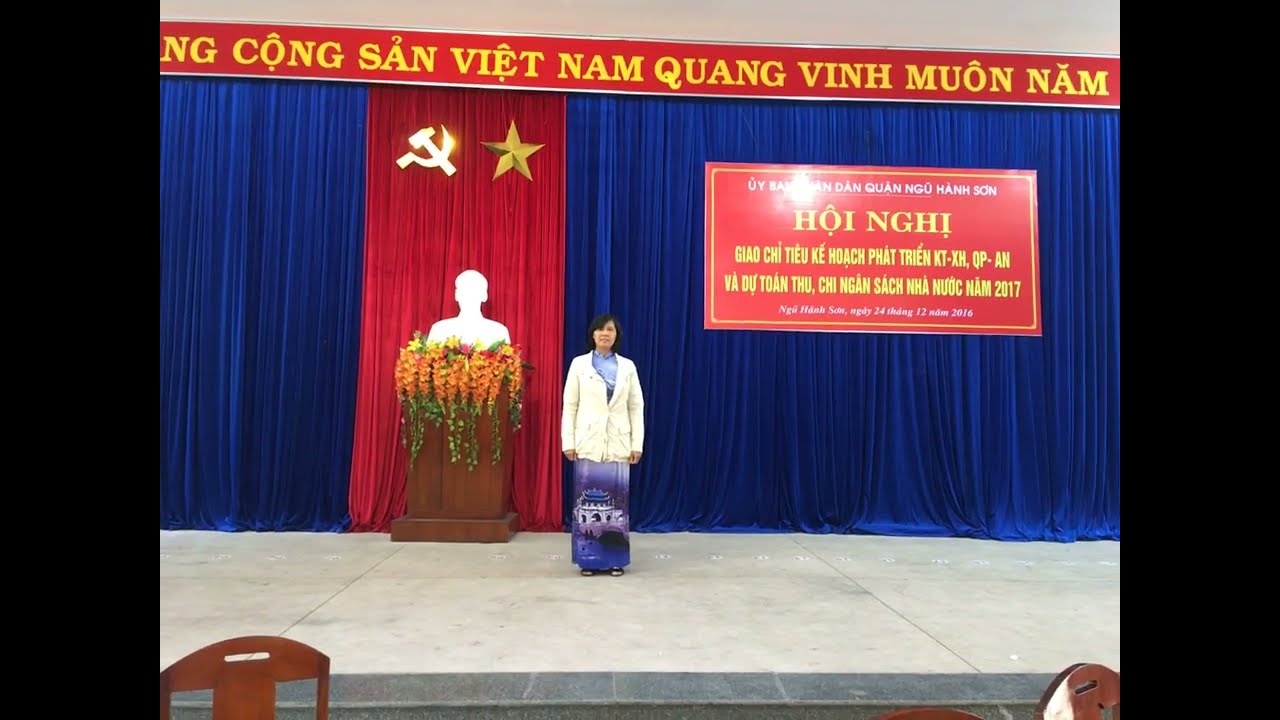The image features a woman standing on a stage with a concrete floor, in the center left, dressed in a white coat and a blue skirt adorned with a detailed design that resembles an old-school Japanese castle. She also seems to be wearing a blue shirt underneath her coat and has short dark hair. The backdrop is a large, elaborate blue curtain with a red section on the left third, prominently displaying communist symbols: a hammer, sickle, and star. Adjacent to her, there is a podium adorned with flowers and a white silhouette of a person. Above her, in the upper right quadrant, hangs a red sign with prominent white letters spelling "H-O-I-N-G-H-I," accompanied by three lines of yellow text beneath it in Vietnamese. The sign additionally mentions the year 2017 in smaller white letters. The setting implies an organized event, possibly a political rally or conference.